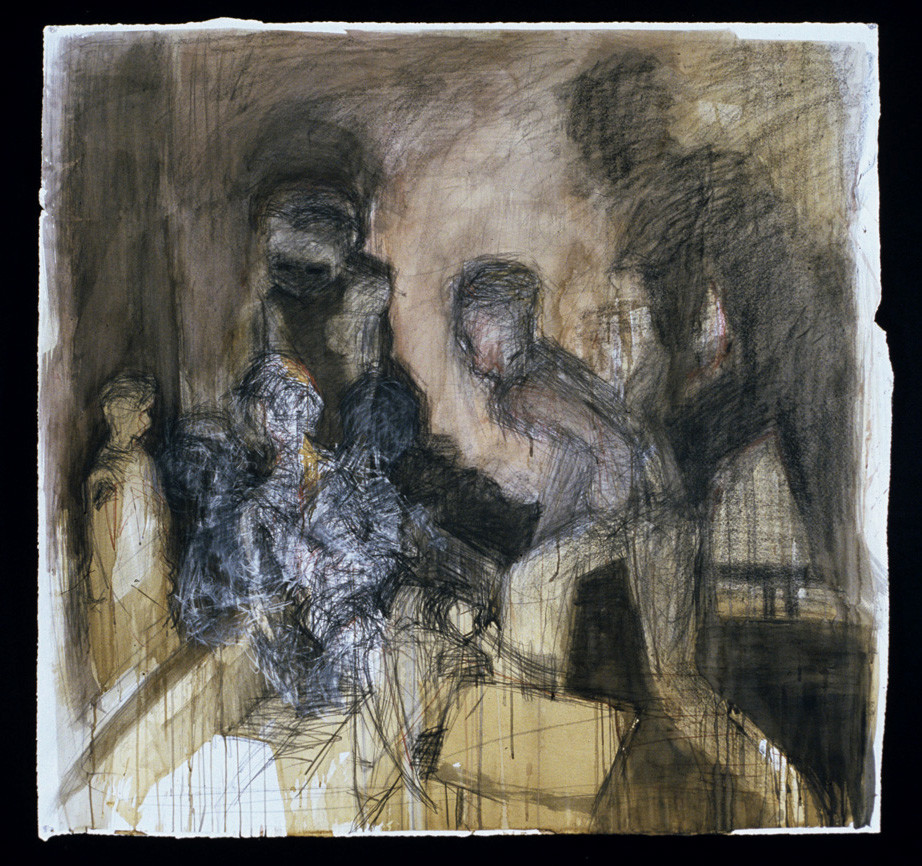The image appears to be an abstract, hand-drawn illustration characterized by a sketchy, rough outline style dominated by a series of lines—both straight and curved. The edges of the image are irregular, resembling torn paper, giving it a raw, unfinished aesthetic. At the center, there is a human figure depicted in predominantly white and tan hues, lying down, possibly on a sofa, suggesting they might be sick or deceased. Surrounding this central figure are four, maybe five other figures, some of which are leaning in, seemingly to inspect or comfort the lying figure. To the right, one figure is leaning forward, their right foot extended, with a shadow behind them. Another figure, possibly female with long orange hair, is looked down upon by a white and gray figure with an alien-like head. On the left, there appears to be a smaller figure, likely a child, illustrated in yellow and white with short hair. The color palette includes tans, browns, whites, blues, yellows, and occasional hints of orange. The background melds these colors together, with notable white areas in the lower left. The overall composition lacks text, numbers, or words, focusing entirely on the interplay of color and line.